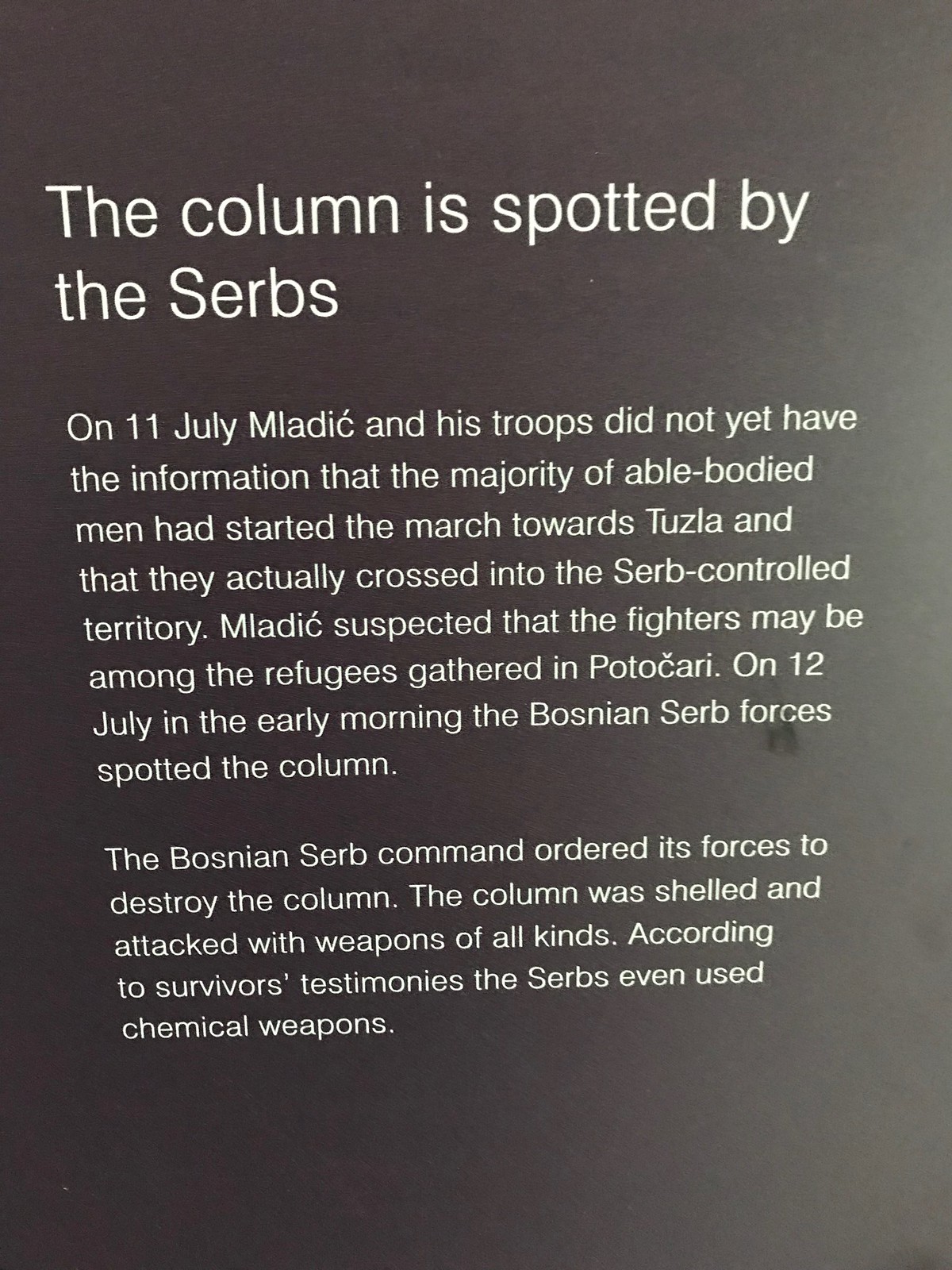This image appears to be of a plaque or a page from a book with a completely black background and white text, detailing a harrowing historical account. The title, prominently displayed in large letters, reads "The Column is Spotted by the Serbs." Below, in smaller letters, the text chronicles the events: On 11th July, Mladic and his troops were not yet aware that the majority of able-bodied men had begun their march towards Tuzla, crossing into Serb-controlled territory. Mladic suspected that some fighters might be hidden among the refugees gathered in Potocari. Then, on 12th July, in the early morning, the Bosnian Serb forces spotted the column. The Bosnian Serb command subsequently ordered its forces to destroy it. The column was shelled and attacked with various weapons, and, according to survivors' testimonies, even chemical weapons were used. The text ends there, abruptly, against the stark black backdrop.